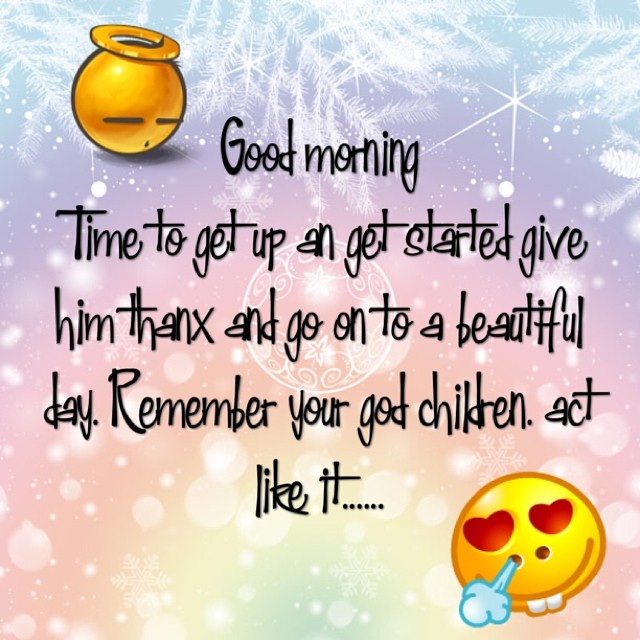The poster is a visually stunning piece with a gradient background that transitions from pale purple to pink, then orange to yellow, creating an ombre effect. Featuring both whimsical and serene elements, the upper portion of the poster is adorned with images of leaves and stars that blend seamlessly into the gradient. The lower section includes subtle, opaque bubbles that add texture to the design. 

In the upper left corner, there's a yellow emoji with an angelic halo, characterized by two thin horizontal lines for eyes and a small dot as a mouth. The lower right corner showcases another yellow emoji, this one with heart-shaped eyes, buck teeth, and steam coming out of its nostrils, giving it a playful expression. 

The central part of the poster carries an inspirational message in elegant cursive script: "Good morning, time to get up and get started. Give Him thanks and go on to a beautiful day. Remember your God children, act like it." The overall effect of the design and typography evokes a sense of calm and motivation, encouraging viewers to start their day positively.